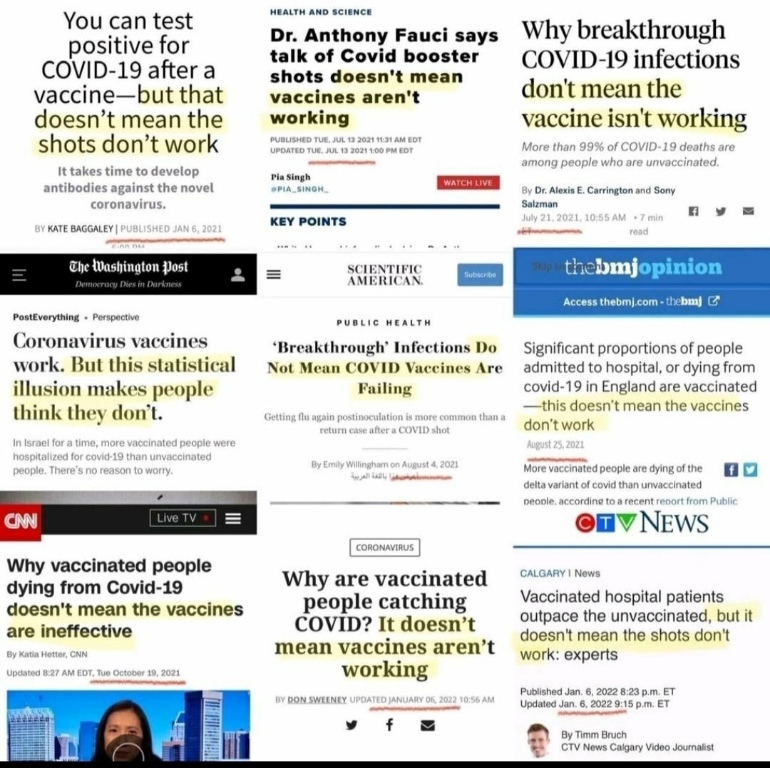The image displays a collage of various headlines arranged in a grid format on a screen. Each headline is encapsulated in a small square and the overall arrangement spans across the frame.

- **Top Left:** "You can test positive for COVID-19 after a vaccine, but that doesn't mean the shots don't work."
- **Top Center:** "Dr. Anthony Fauci says, talk of COVID booster shots doesn't mean vaccines aren't working."
- **Top Right:** "Why breakthrough COVID-19 infections don't mean the vaccine isn't working."
- **Middle Left:** "Coronavirus vaccines work, but the statistical illusion makes people think they don't." (Washington Post)
- **Middle Center:** "Breakthrough infections do not mean COVID vaccines are failing."
- **Middle Right:** "Significant portions of people admitted to hospital or dying from COVID-19 in England are vaccinated. This doesn't mean the vaccines don't work."
- **Bottom Left:** "Why vaccinated people dying from COVID-19 doesn't mean the vaccines are ineffective." (CNN)
- **Bottom Center:** "Why are vaccinated people catching COVID? It doesn't mean vaccines aren't working."
- **Bottom Right:** "Vaccinated hospital patients outpace the unvaccinated, but it doesn't mean these shots don't work."

Overall, the captions collectively highlight a common theme: despite breakthrough infections and the occurrence of COVID-19 cases among vaccinated individuals, vaccines remain effective.